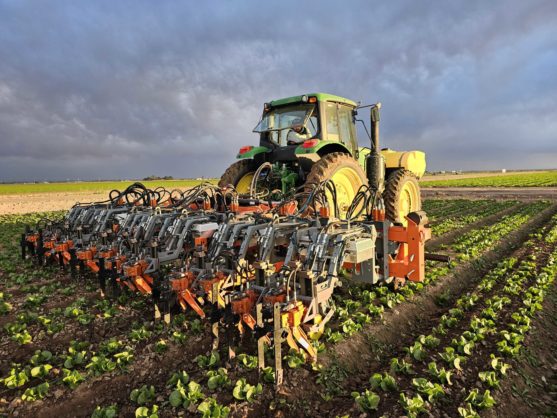The image is a detailed photograph of a large, expansive farm, featuring multiple neat rows of green plants with small furrows in between, stretching into the distance. At the far edge of the field, a line of trees marks the boundary, beyond which dark gray mountain ranges loom under a sky that transitions from a clear light blue at the top to clouds that resemble strands and fog near the horizon. Central to the image is a robotic, boxy, orange farming machine with no cockpit or driving cab, supported by four large black wheels and equipped with a significant orange contraption on its back. Walking behind this automated equipment is a person wearing blue jeans, a black cap, and an orange and yellow safety vest, seemingly controlling the machine with a device in their hands.